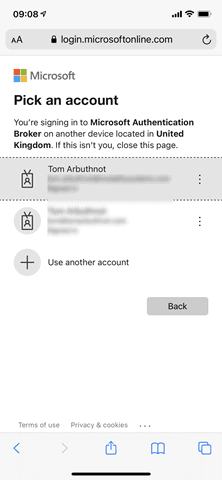This image captures a screenshot of a smartphone displaying the Microsoft Online login page. It was taken at 9:08 AM, as indicated by the timestamp at the top of the screen. The device shows full Wi-Fi connectivity and a fully charged battery. The login interface prompts the user to pick an account from a list of several options, although much of the personal information, like account names, is obscured or redacted for privacy. The overall screen appears routine and lacks eye-catching details, emphasizing its utilitarian nature as a secure sign-in portal.